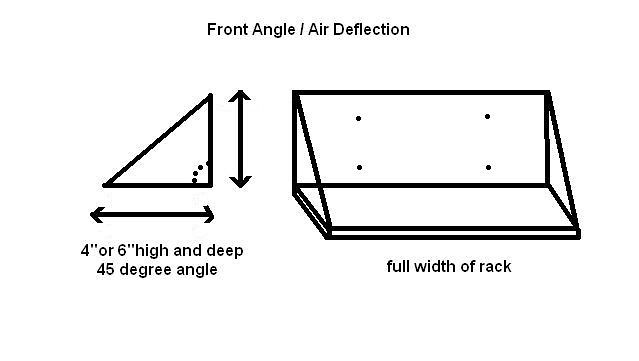The image is a detailed black-and-white technical illustration, possibly hand-drawn or computer-generated, providing design instructions for a wall-mounted rack. At the very top, centered in black typed text, it reads "Front Angle/Air Deflection" with capitalized "Front," "Angle," "Air," and "Deflection," while the remaining letters are in lowercase. 

On the left side of the image, there is a prominent triangle, positioned with its long side on the left, giving it the appearance of leaning on its side. This triangle is detailed with double-sided arrows: one arrow runs horizontally along the base indicating "4 inch or 6 inch high and deep" with a 45-degree angle, while another arrow runs vertically, defining the height of the side. The right angle of the triangle is marked with four small dots in a roundish pattern.

To the right of the triangle, the illustration features an angular depiction of the rack, referred to as a triangular prism, with clear black outlines. Below this, a label reads, "Full width of rack," indicating this component's span from left to right. The drawing illustrates the rack's side profile extending out from the wall, with four screw holes depicted for mounting purposes. All elements of the illustration – text and drawings – are rendered in black against a white background.